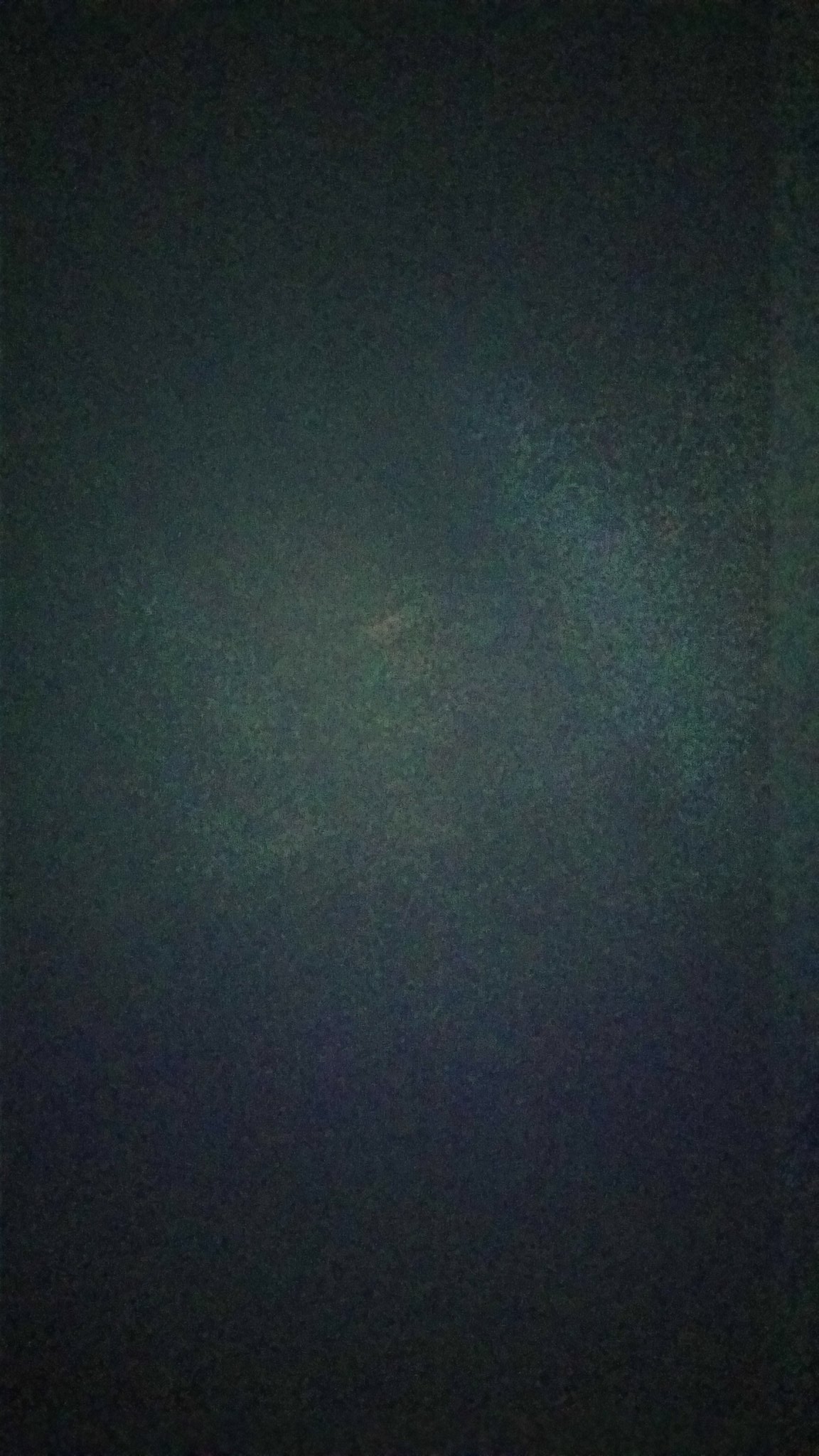This photograph, though low in quality, presents an intriguing display of colors despite its graininess and underexposure. The image primarily consists of muted hues that resemble the iridescent reflection of a peacock feather, yet it remains abstract with no discernible objects. Dominating the center is a vertical streak of blue alongside an orangish-yellowish-green streak, lending the composition a streaky, painterly quality. Speckled blue dots faintly appear below this vibrant core, adding subtle texture. The photo appears to have been captured through textured glass, which contributes to its disjointed, pixelated appearance and elongated vertical crop. The overall palette is dominated by dark shades, ranging from black to various grays, enhancing the moody and enigmatic nature of the image. It exudes an accidental yet curious charm, emphasizing the unpredictable beauty found in unintended moments.